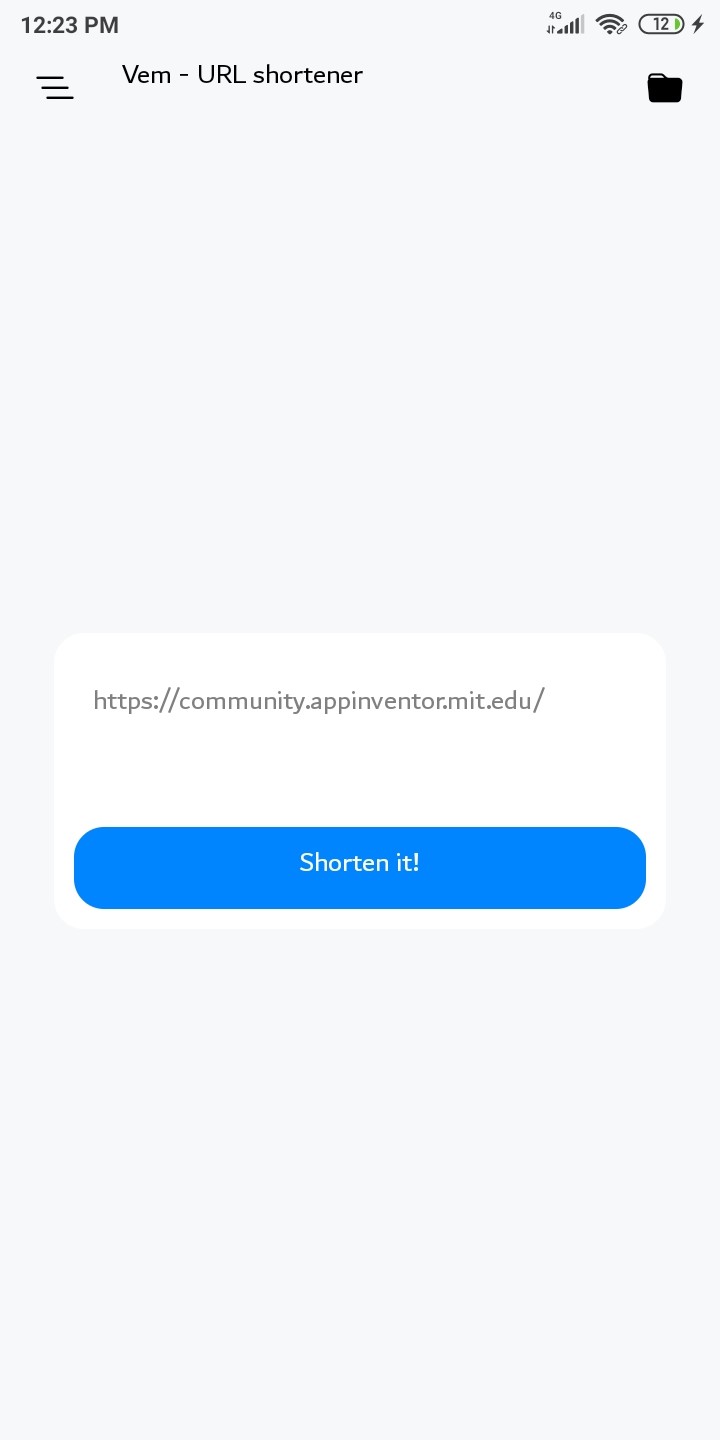The image displays a smartphone screen showing an app interface for a URL shortener. At the top of the screen, the status bar reveals the current time as 12:23 PM. Adjacent to the time are various icons, including a Wi-Fi symbol, a cellular signal indicator, and a battery icon showing 12% with a charging symbol.

Beneath the status bar, the app's header features the title "VEM, URL Shortener," accompanied by a black file folder icon. On the same line, to the right, there are three horizontal black lines representing the settings menu.

Located further down on the screen is a white text box containing a URL: https://community.appinventor.mit.edu/. Below this box, there is a blue button labeled "Shorten!" in white text, indicating the function to shorten the URL.

The overall background of the app interface is a subtle gray, creating a clear contrast with the darker text and icons. The screen is typical of a smartphone interface, with most of the content displayed in black and gray text, accented by a few colorful elements, such as the blue "Shorten!" button.